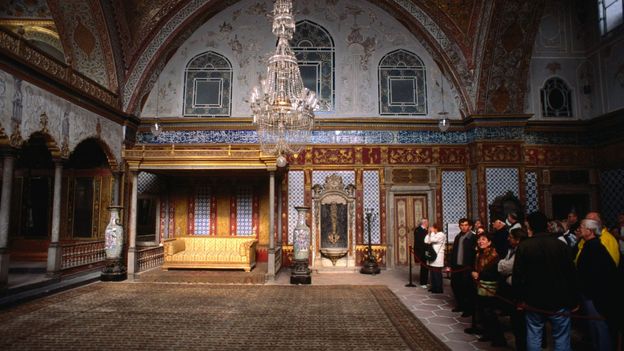The photograph captures the interior of an ornate, likely historic mansion. Dominating the center of the image from the top is a large, intricate crystal chandelier hanging from the vaulted ceiling, which features arch shapes and possibly weathered wallpaper or patterned decor. The room boasts high ceilings and expansive windows with curved arches at their tops. On the left-hand side, a golden-yellow couch is prominently featured, flanked by tall decorative vases on pedestals. A large, brown and tan rug lies atop hexagon-shaped tiles that span the flooring. In the bottom right quadrant, a crowd of people stands behind a rope barrier, seemingly on a guided tour, dressed in long-sleeve jackets and shirts as if it's a cool day. The grandeur of the room, with its detailed furnishings and architecture, suggests it is a popular attraction for visitors.